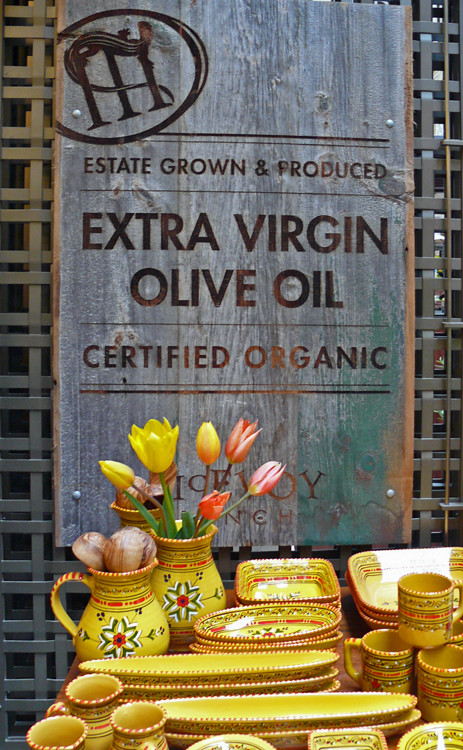The photograph showcases an assortment of bright mustard yellow dishware arranged on a table, including oval bowls, long bread-shaped bowls, mugs, square plates, and pitchers. Each piece is adorned with a floral design, intricate repeating patterns, and delicate brown and white striped rims, giving them a handcrafted and potentially Indian aesthetic. A pitcher filled with fresh tulips adds a touch of natural beauty to the display. This extensive collection suggests the items are likely for sale rather than part of a personal set. Behind the table, a gray wooden sign with a wood-grain texture is mounted on a thick metal mesh grid. The sign features an emblem resembling an 'M' with a swirl, followed by the inscriptions: "Estate Grown and Produced," "Extra Virgin Olive Oil," and "Certified Organic." The natural and bright lighting gives the impression that the photo is taken indoors, possibly in a well-lit market or store setting.